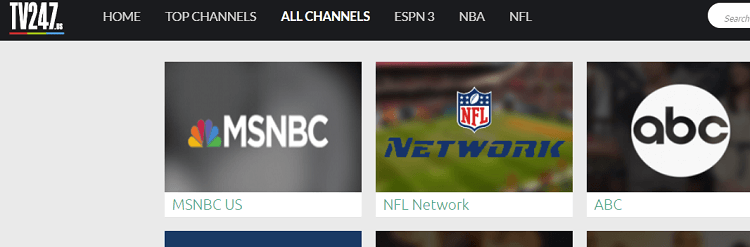This image is a screenshot from the TV247 website. In the upper left-hand corner, there is a prominent logo that reads “TV247” in uppercase letters, using a consistent white font size. Directly below the logo, a thin horizontal bar appears, featuring a gradient of red, yellow, and blue colors. This bar sits atop a blue menu bar that spans the width of the image. Above this, there is an additional black bar that also runs horizontally across the screen.

The menu bar contains several navigation options, all in white text. These options, listed from left to right, are: "Home", "Top Channels", "All Channels", "ESPN3", "NBA", and "NFL". Below this navigation menu, three distinct buttons are visible. The first button is for MSNBC, identifiable by the iconic peacock symbol, followed by the text "MSNBCUS" written in a white rectangle with green font. Next, there is a button for the NFL Network, and lastly, a button for ABC.